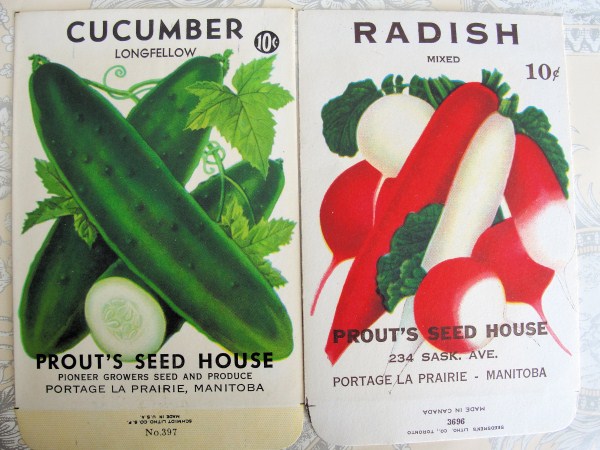The image displays two seed packets side-by-side, both with white backgrounds. The left packet is labeled "Cucumber Longfellow" at the top, with a price tag of 10 cents indicated by a black circle with white numbers in the upper right corner. It features a picture of three dark green cucumbers, two arranged in a crisscross pattern and one sliced open to display its interior. There is also a small vine with two green leaves. At the bottom, the packet is marked "Prouts Seed House, Pioneer Growers Seed and Produce, Portage, La Prairie, Manitoba."

The right packet is labeled "Radish Mixed" and priced at 10 cents. The image on this packet shows a variety of radishes, some red and some white, with different shapes including long and round. Green leaves are scattered around the radishes. At the base of the packet, it reads "Prouts Seed House, 234 Sask Avenue, Portage, La Prairie, Manitoba." Both packets emphasize the origins and detailed branding from the seed company.